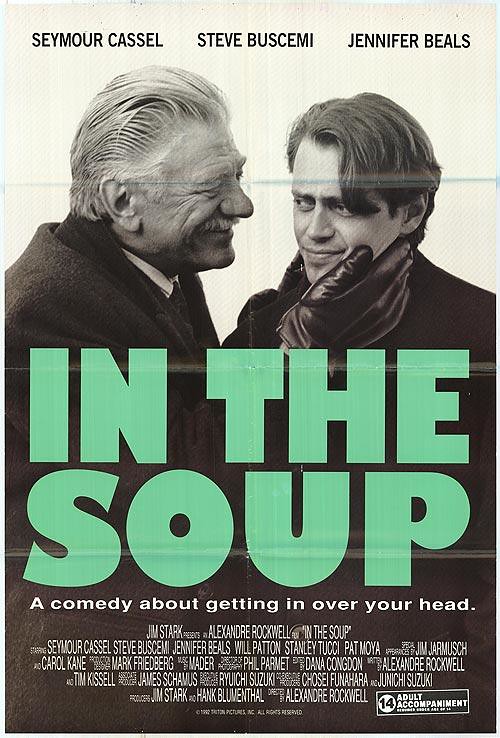The image is an advertisement for the movie "In the Soup," prominently showcasing its title in large green text just below the center line of the poster. At the top, the poster lists the film's stars: Seymour Cassel, Steve Buscemi, and Jennifer Beals. Primarily in black and white, the poster features a scene where an older actor in a suit, tie, and gloves, likely Seymour Cassel, is playfully tapping the cheek and jaw of a younger Steve Buscemi, who is depicted with long hair and a grimacing expression. The tagline beneath the title reads, "A comedy about getting in over your head." Additional credits for the director and other contributors are present at the bottom in small print. The poster also indicates that the movie is meant for viewers aged 14 and older, suggesting an older release date possibly from the 70s or early 80s, especially given Buscemi's notably youthful appearance.